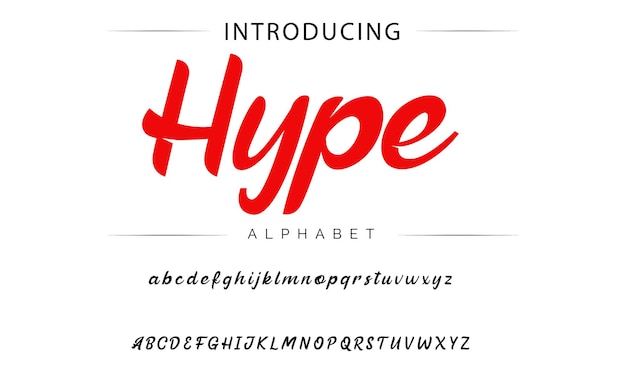The image features a promotional advertisement for a new font called "Hype." Set against a clean, all-white background, the design is meticulously structured. At the top, the word "INTRODUCING" is displayed in black, uppercase letters, flanked by thin gradient lines on either side, giving it a banner-like appearance. This header is followed by the word "HYPE," prominently showcased in large, red calligraphy with a capitalized "H," making it the focal point of the image. Below "HYPE," the word "ALPHABET" appears in smaller, all-uppercase black text, also bordered by similar gradient lines. The lower section of the image is dedicated to illustrating the "Hype" font in detail: first, with the alphabet presented in all lowercase letters from A to Z, and then repeated in uppercase, both sets rendered in the black, cursive-like font style of "Hype." The characters maintain a cursory flow without being connected, emphasizing the unique aesthetics of the font.